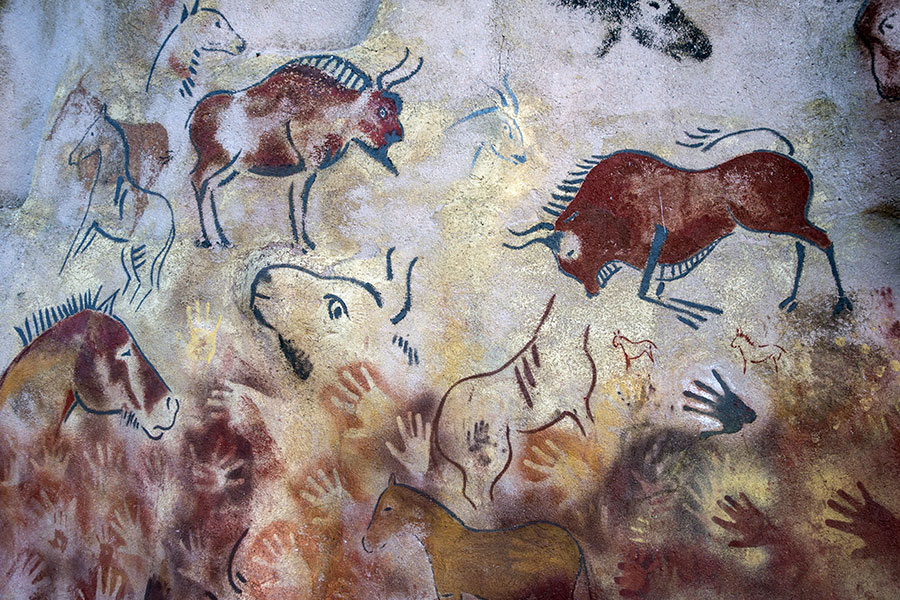The image, resembling primitive cave art, features a horizontally aligned rectangular panel with a stone-like, grayish background textured with smudges of brown and blue. The top section showcases multiple animal figures: on the upper left, there is an outline of a horse in blue, with a horse's head above it. Next to these is a larger figure with blue legs and a brown body, adorned with horns, possibly depicting a bull or elk. This animal is intricately shaded in brown and gray. On the right side, there's another similar figure facing left, also with brown shading and blue lines that suggest movement, as if the animal is running.

Transitioning to the browner background at the bottom, the image is filled with a multitude of handprints in various shades of brown and blue, both positive (filled-in) and negative (spray-painted silhouettes). Among these handprints, on the lower left side, is another horse's head with a blue mane and a face shaded in white and brown. The two-dimensional art style conveys a sense of antiquity, whether genuinely ancient or a modern attempt to replicate the aesthetic of ancient cave paintings.